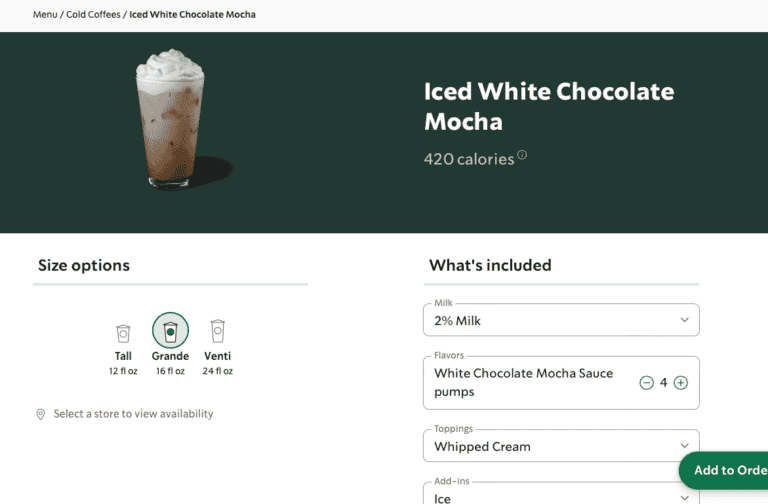The image showcases a detailed coffee order menu on a white background. At the very top, there are main menu options listed horizontally: "Menu," "Cold Coffees," and "Iced White Chocolate Mocha." The upper third of the screen features a dark green background with an enticing image of an iced coffee drink in a clear glass, topped with whipped cream. The drink is labeled "Iced White Chocolate Mocha" with a notation of "420 calories" in white font beneath the name.

In the lower two-thirds of the screen, the left side displays three size options, each represented by a cup icon. The options are "Tall" (12 ounces), "Grande" (16 ounces), and "Venti" (24 ounces), with the "Grande" size selected and highlighted by a green circle. Below the size options is a prompt to "Select a store to view availability."

On the right side, there are customizable drink options under the heading "What’s Included." The first option, "Milk," has a dropdown menu where 2% milk is selected. The next option, labeled "Flavors," allows for the adjustment of the "White Chocolate Mocha Sauce" by using plus or minus signs, currently set at four pumps. The third option deals with "Toppings," with whipped cream selected from a dropdown menu. The last option, "Add-Ins," shows ice as the chosen add-in, also with a dropdown menu.